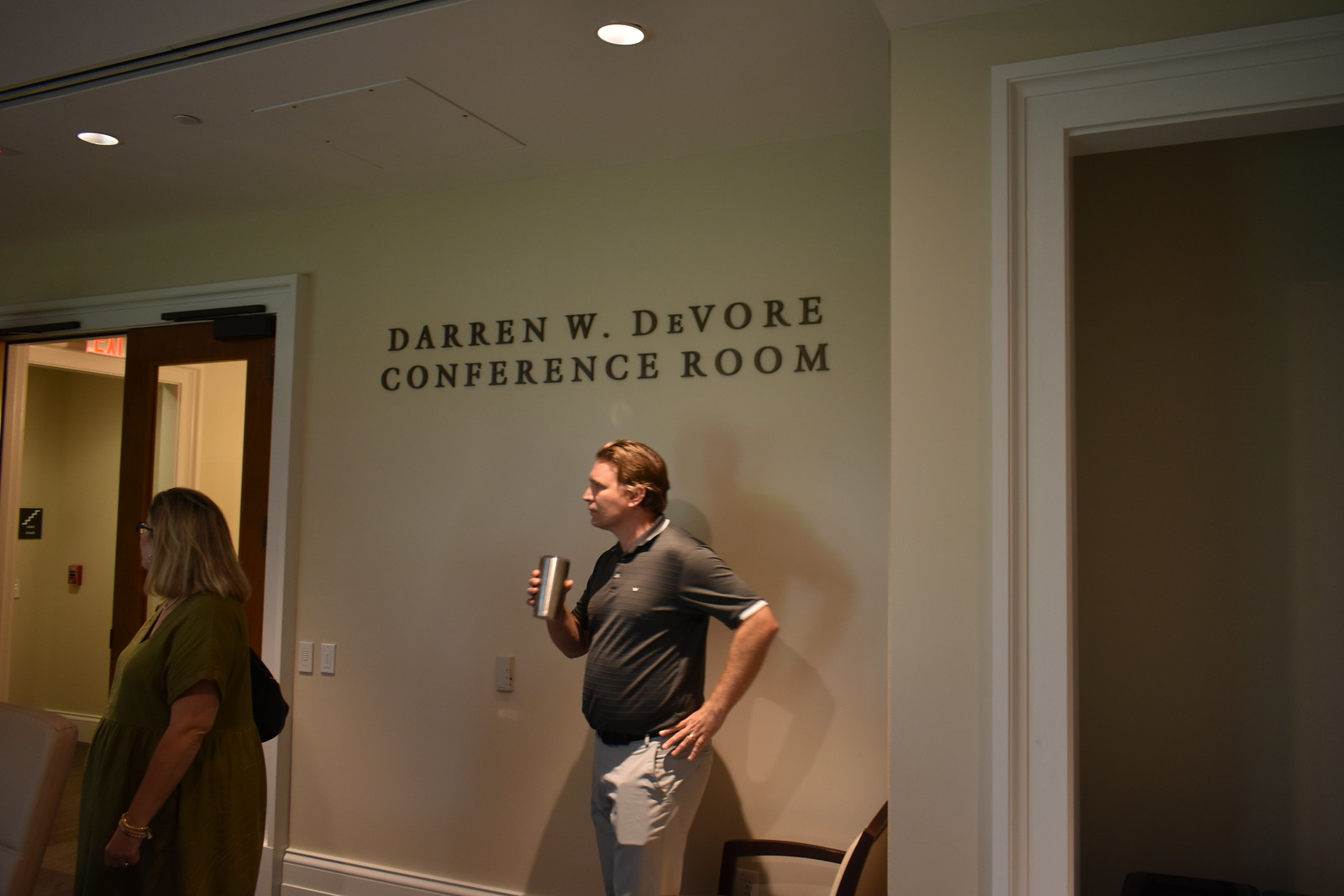In the image, we see an indoor setting which appears to be a conference room. The room is illuminated by recessed lighting from the ceiling, casting a soft light on the scene. Dominating the center of the image, a man of Caucasian descent with brown hair stands facing towards the left. He is dressed in a short-sleeve gray polo shirt and light gray khakis. His left hand is positioned on his hip while his right arm, bent at the elbow, holds a stainless steel tumbler. He stands directly beneath a black sign on the tan-colored wall that reads "Darren W. DeVore Conference Room."

To the left of the man, there is a set of double doors framed by white molding. The door to the left is open, revealing a glimpse of another hall and an exit sign, leading to what appears to be emergency stairs, while the door to the right remains closed. In the lower left part of the image, a woman of Caucasian descent with shoulder-length straight blonde hair and glasses is also facing left, thereby obscuring her face. She is wearing a long, loose-fitting green sundress and appears heavier set. 

On the right-hand side of the image, there is another open doorway with a similar white molding, leading into a longer hallway. A few chairs are scattered around the room, enhancing the typical conference room setting. The photo is rectangular, wider than it is tall, capturing the detailed arrangement of the room and its occupants. The wall colors range from white and tan to off-green gray, adding a muted palette to the overall image.